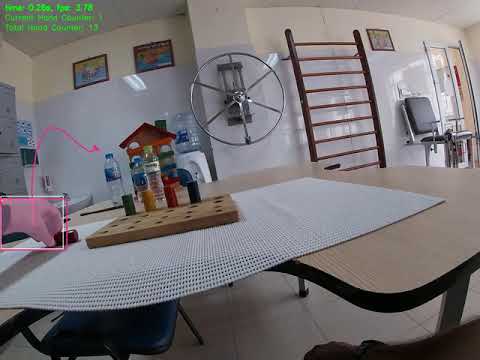The image depicts an indoor setting that appears to be a restaurant with a nautical theme, suggested by a silver ship's wheel and a captain's chair visible on the right-hand side. In the center of the table, there are condiments resting on a distinctive net-webbed surface that suggests a maritime ambiance. A person's left hand is reaching out, making contact with a black object on the table. This hand is enclosed within two bounding boxes – a pinkish one and a white one – indicative of pattern recognition or augmented reality software in use. 

A pink line extends from the top of the fist, curving slightly to the right and extending toward the back wall, marked by a whiteboard. The upper left corner of the image features green text, split into three lines, though it is too blurry to be legible. The table also holds various objects including a small toy that requires filling with shapes, a filter-like white sheet with tiny squares, and a row of four water bottles that are different in colors – two are bluish, one is clear, and one is a darker grayish-blue.

The background reveals additional elements: a toy house and a water container bucket behind the bottles; a vertical rectangular casing behind a silver circle wheel; and a wooden ladder for exercise, about four feet wide and eight feet tall, to the right of the scene. Adjacent to this, a swivel chair is positioned near a set of glass doors, with one door open on the right end. The upper left corner of the image also contains two pictures and unreadable information, possibly from a website.